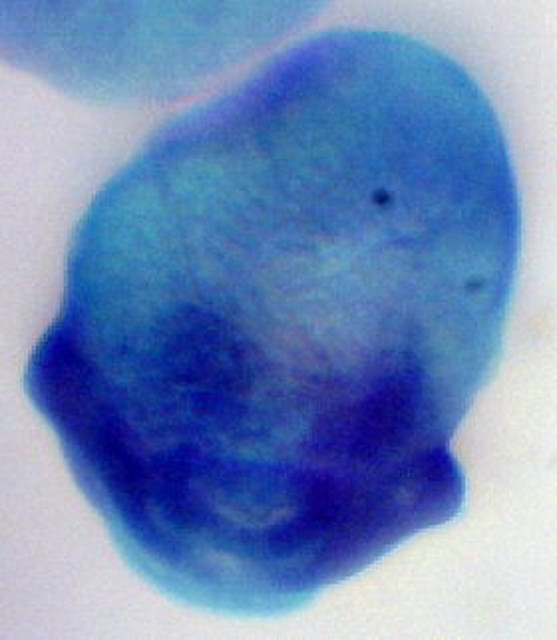The image appears to be a highly magnified view of an amoeba-like structure, prominently showcased as a large blue blob with a distinct oval shape. The specimen is characterized by two small black dots resembling eyes, and its coloration transitions from a lighter blue at the top to a darker blue at the bottom, suggesting a diffusion gradient of some sort. The background is a stark white, providing contrast that accentuates the structure. The blob, with its fuzzy outline, seems almost anthropomorphic, reminiscent of an alien head due to its potato-like shape and the positioning of the dots as eyes. The rectangular, vertically oriented picture has a slightly hazy quality, reinforcing the idea that it is an image viewed under a microscope, potentially in a scientific setting such as a classroom or laboratory presentation.